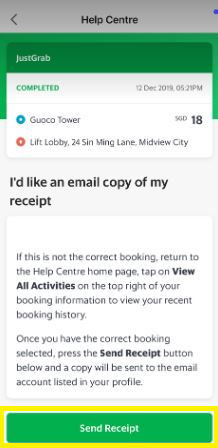This image is a screenshot of a phone displaying a section of the Help Center. The top part of the screen features a gray banner with a back arrow, and in the center, the words "Help Center" are displayed in black text. Below the banner, there are two green bars; the top bar reads "just grab" in white letters, and the lower green text states "Completed December 2019, 5:21 PM."

Beneath these bars, there is a white area labeled "Completed". On the left side within this section, there is a blue icon and next to it, the text "Guaco Tower." Below this, there is a red icon to the left that accompanies text detailing "Lip Lobby, 24 Sin Ming Lane, Midview City" and to its right, albeit a bit blurry, it appears to say "6D." Further to the right in bold black text is the number "18".

Continuing downward, there is a bolded text in gray that states in large letters: "I would like a copy email copy of my receipt." Following this, an instruction reads: "If this is not the correct booking, return to the Help Center home page." Additional instructions underneath advise users to "Tap on view all activities (or view AH activities, it’s a bit blurry) at the top right of your booking information to view your recent booking history. Once you have the correct booking selected please press the send receipt button below and a copy will be sent to the email account you listed on your profile."

At the bottom of the page, there's a large, dark green button with a yellow outline that says "send receipt" in white text.